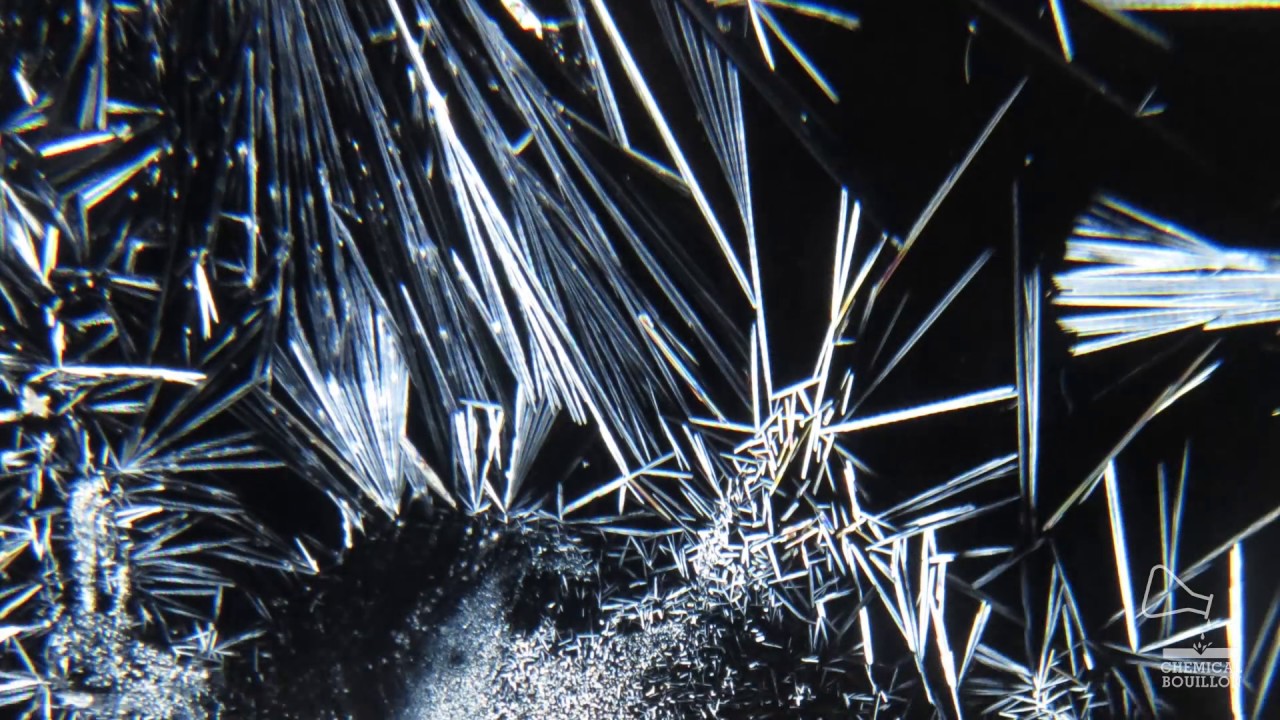The image under the microscope reveals numerous tiny shards that resemble either glass or metallic shavings, scattered against a black background. These shards are iridescent and possess a shiny, reflective quality, ranging in size from long, spiky strands to very short fragments, some as tiny as ants. Their clear, silver-like appearance and varied arrangement give them a crystalline, almost ethereal look. In the bottom right corner of the photo, there's a transparent logo of a flask, turned on its side with a drop falling from it, accompanied by small letters that read "CHEMICAL BOLO."